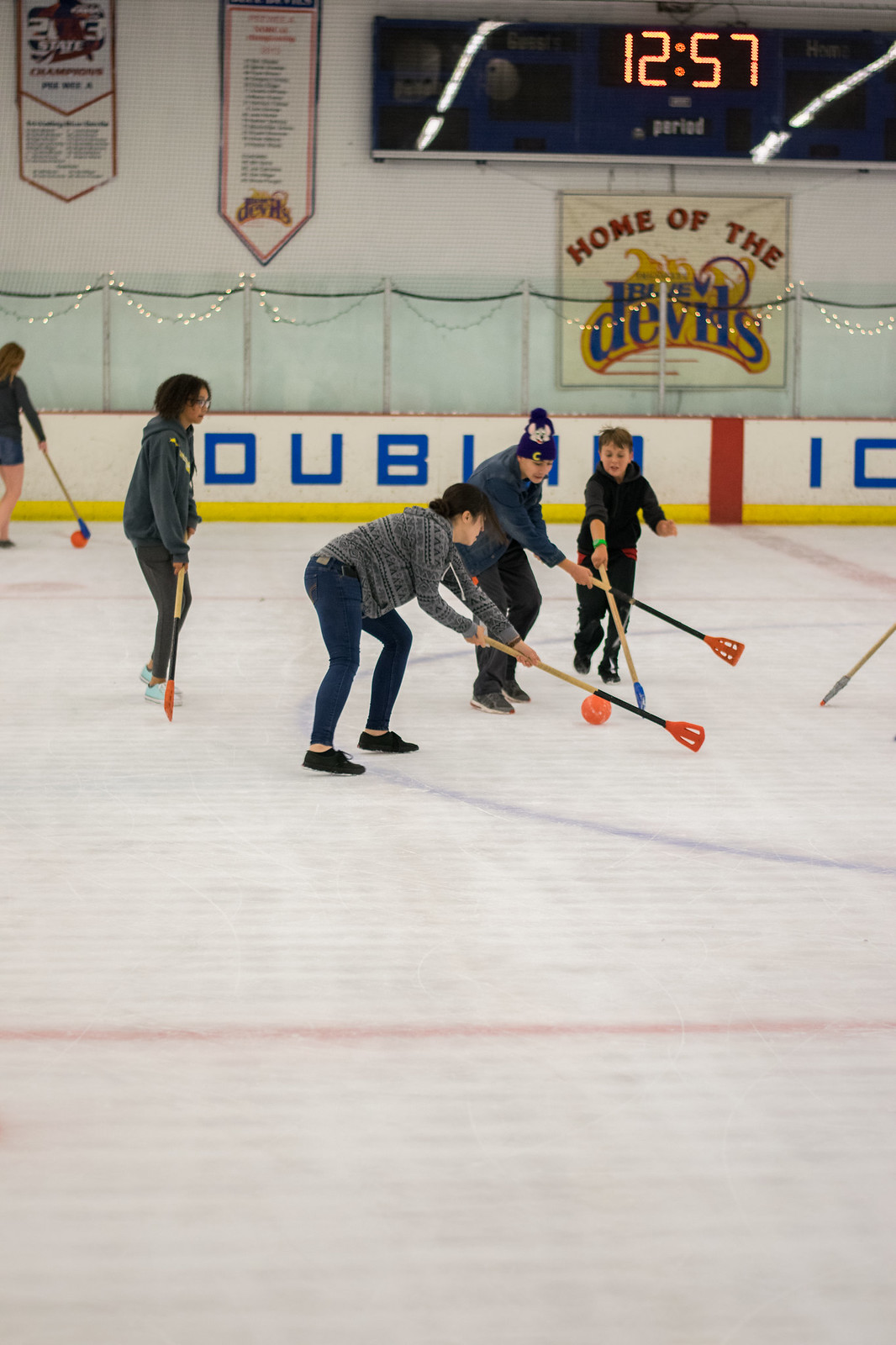The image captures an ice hockey rink scene featuring a group of young teens, likely in their early teens, playing a casual game of floor hockey or a similar hockey derivative. They are dressed in casual clothing with regular sneakers instead of ice skates and are using wooden and plastic sticks to play with an orange ball. In the center of the rink, three players are vying for the ball: a young girl on the left and two young boys on the right, with one boy reaching out closest to the ball. Another young girl is positioned behind these three, further back on the ice. In the background, to the left, another player with a stick can be seen, also handling an orange ball. On the extreme right of the image, there is a stick lying on the rink.

The rink is marked with red and blue lines and features writing along the boundary wall that spells out "D-U-B," likely shorthand for Dublin. Prominent on the far wall is a square banner reading "Home of the Devils" in red and blue lettering, complemented by a scoreboard displaying the time "12:57." The top right corner of the rink wall is adorned with various banners, and festive lights are strung along the transparent glass barriers enclosing the rink.